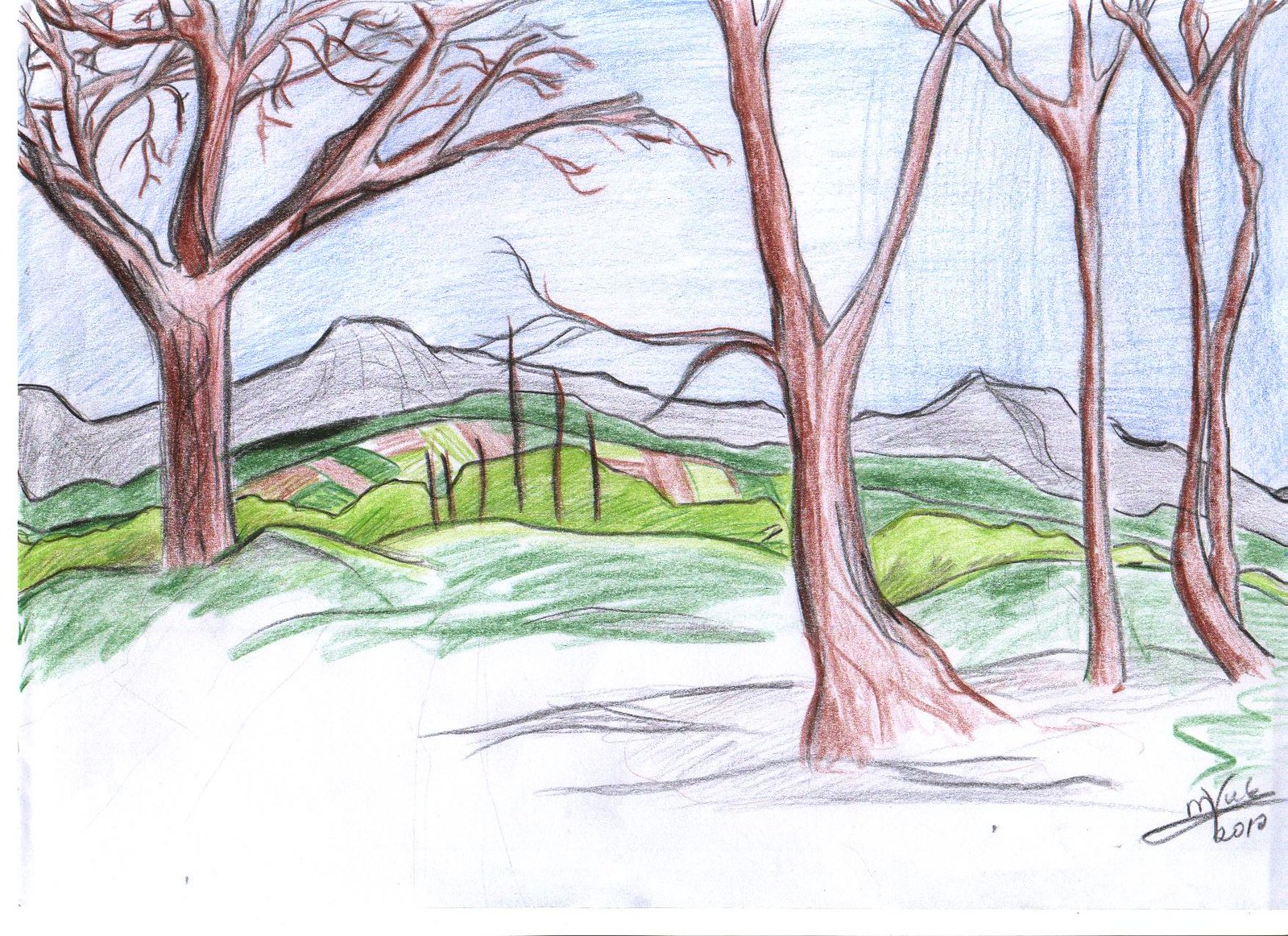This detailed sketch portrays a serene outdoor setting featuring four distinct trees and various undulating hill structures. On the bottom right corner, the artist's signature along with the year '2012' is inscribed in black text. 

The sketch starts at the bottom with a white-colored ground, transitioning into a cluster of three tree bases situated on the right-hand side. These trees are minimally detailed with few branches. In contrast, a larger tree dominates the left-hand side, characterized by a trunk that splits into three major branches, each adorned with numerous smaller offshoots.

Behind the trees, the scene unfolds with shades of light green, accented by patches of pink and green, transitioning into a series of green and gray mountaintops. The backdrop is completed with a sky at the top of the sketch, beautifully shaded in hues of white and blue. This harmonious blend of natural elements creates a peaceful and captivating landscape.